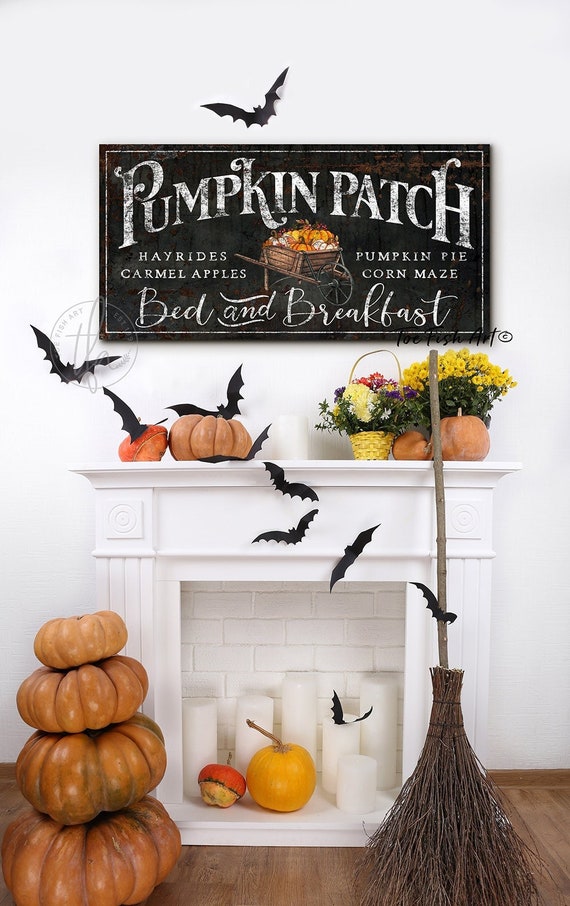The image portrays a cozy, fall-themed living room with a prominent white fireplace as the focal point. The fireplace, adorned with detailed crown molding, stands against a matching white wall and wooden floor. To the right, an old-style witch's broomstick with a decorative bat leans against the mantle. 

The mantle hosts a festive array of fall decorations, including chrysanthemums, colorful gourds, and decorative pumpkins. Above the mantle, a rustic black sign with white lettering lists autumnal delights such as "Pumpkin Patch, Hay Rides, Caramel Apples, Pumpkin Pie, Corn Mazes, Bed and Breakfast." The sign features an illustration of a wheelbarrow filled with pumpkins, enhancing the seasonal atmosphere. 

Scattered throughout the scene are black construction paper bats, adding a touch of Halloween spirit. Inside the fireplace, where a fire would typically burn, six white pillar candles, a medium-sized yellowish pumpkin, a small orange pumpkin, and another decorative bat create a warm and inviting display. On the lower left side of the image, a stack of four graduated plastic pumpkins, resembling a snowman, completes the charming fall decor.